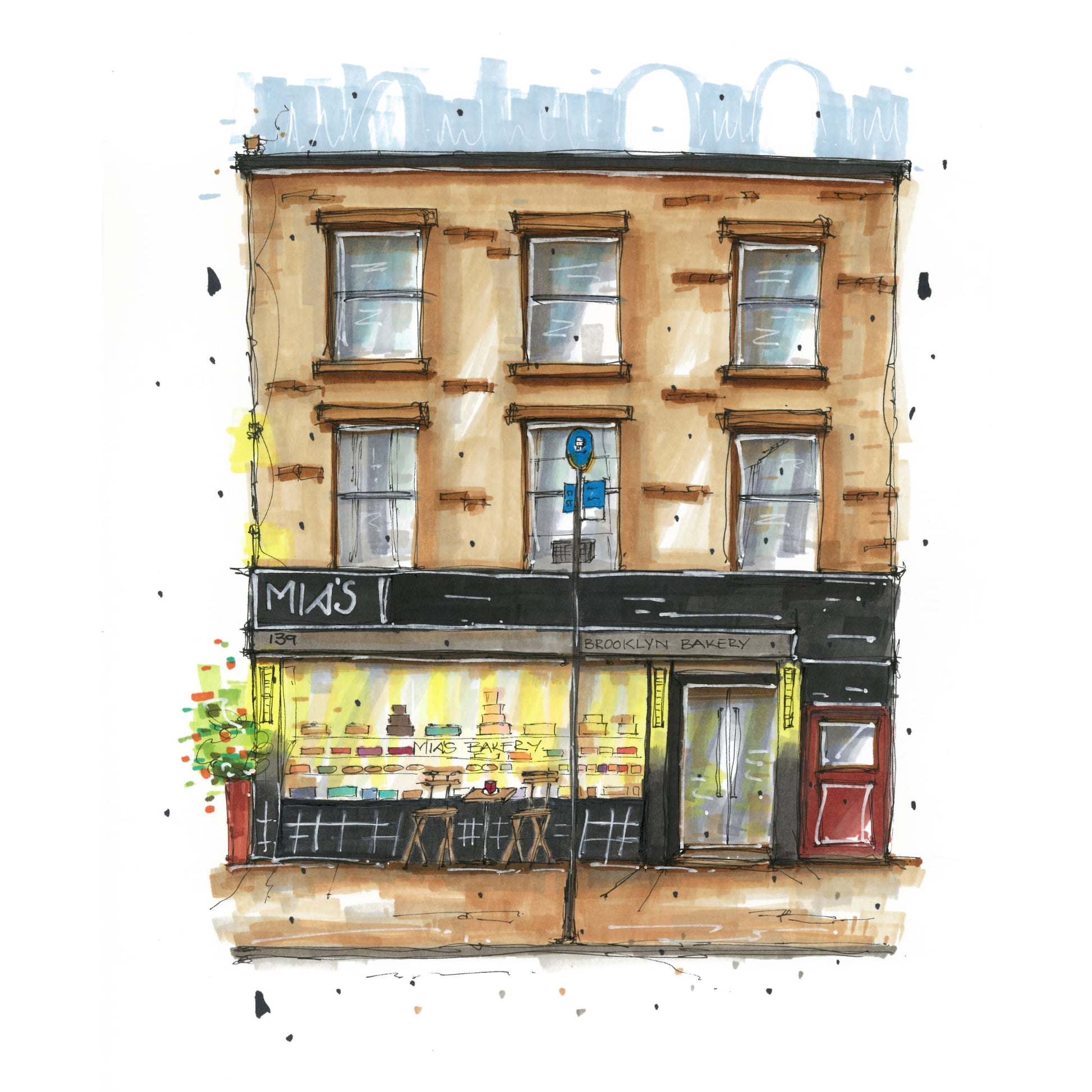This is a detailed marker drawing of a brownstone-style building, characterized by its tan and dark brown brickwork. The ground floor houses Mia's Brooklyn Bakery, prominently marked by a black rectangular sign with "Mia's" in white lettering and a gray sign below reading "Brooklyn Bakery." The bakery features a large glass window displaying roughly sketched pastries on various shelves inside. On the right, double glass doors serve as the main entrance, and to the left, a red door likely leads to the apartments above. The sidewalk in front of the bakery includes two chairs and a small table, creating a quaint outdoor seating area. A lamppost stands nearby, and a small tree adds a touch of foliage to the scene. The upper levels of the building consist of two stories with a total of six double-paneled windows, each adorned with large windowsills, suggesting residential apartments above the bakery.